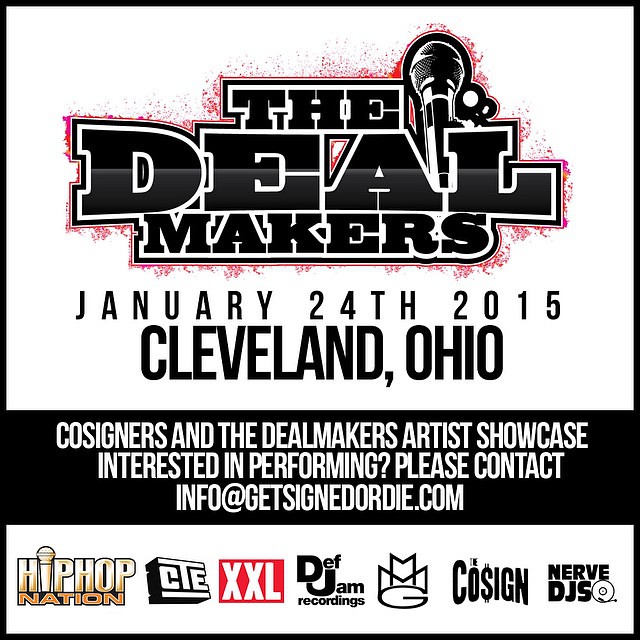This advertisement poster, primarily in black and white with touches of red and yellow, promotes an event hosted by The Dealmakers taking place on January 24th, 2015, in Cleveland, Ohio. The poster features a decorative logo for The Dealmakers in large black letters with a pink border, positioned at the top. Below this, the date and location are clearly stated. A black strip across the middle highlights the core message in white letters: "Co-signers and The Dealmakers Artist Showcase. Interested in performing? Please contact info at GetSignedOrDie.com." The bottom section of the poster, set against a white background, displays the logos of several sponsors, including Hip Hop Nation (with yellow at the bottom of their logo), CTE (white letters on a black background), XXL (with a red outline), Def Jam Recordings, MMG, The Co-sign, and Nerve DJs. A drawing of a microphone is also present to the left, just above the event details.